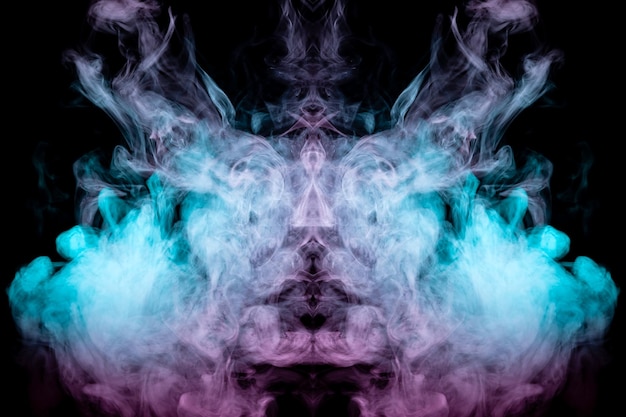The image features a striking symmetric composition against a solid black background that is slightly wider than it is tall. A vibrant display of smoky patterns dominates the center, reminiscent of cotton candy colors—rich magenta, sky blue, and shades of white swirl together seamlessly. The smoke shapes a captivating mirror image on both sides, with the left side mirrored exactly by the right. Emerging through the luminous wisps of smoke, a central statue-like figure stands out with striking angularity. The figure is adorned with two prominent horns at the top, leading down into a lateral diamond shape, with indents suggesting eyes and a mouth. Its body continues downward, highlighted by a diamond on its chest and a triangle near where a waist would be. The interplay of colors gives the impression of white smoke at the forefront, surrounded by blue and greenish-blue hues near the center, and transitioning into a purplish glow towards the base, all beautifully framing the enigmatic central figure.